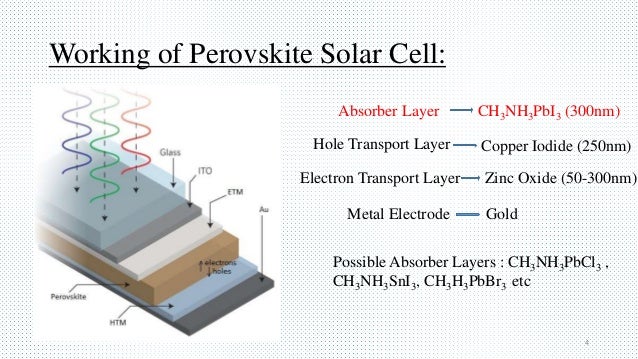This image is a detailed diagram of a perovskite solar cell titled "Working of a Perovskite Solar Cell," with the title prominently underlined at the top. The diagram is placed on a white background adorned with light black dots, enhancing its visibility. The left side of the page features a color-coded, layered representation stacked with labels: Glass, ITO, ETM, Perovskite, HTM, and AU (gold), each identified with arrows. This illustration depicts various layers in blue, dark gray, light cement, brown, light blue, and dark gray. Squiggly lines in dark blue, green, and red run vertically above the layers. 

On the right side, centered text in both red and black provides further details: 
- "Absorber Layer - CH3NH3PbI3 (300 nanometers)" in red
- "Hole Transport - Copper Iodide (250 nanometers)" in black
- "Electron Transport Layer - Zinc Oxide (50 to 300 nanometers)" in black
- "Metal Electrode - Gold" in black  

Below this section, additional potential absorber layers are listed, including:
- "CH3NH3PbCl3"
- "CH3NH3SnI3"
- "CH3NH3PbBr3," among others.